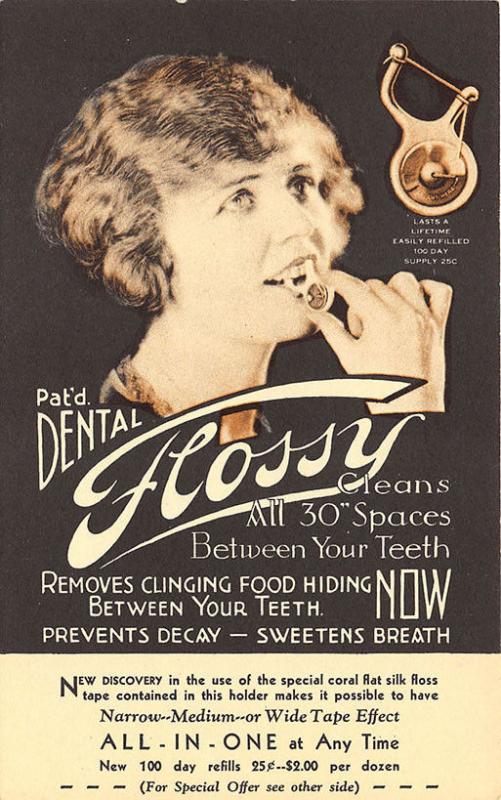The image is a vintage poster advertisement for dental floss, likely from the 1950s, based on the font, woman's hairstyle, and design elements. It features a woman smiling as she uses an old-fashioned dental floss, which appears to be attached to a holder for ease of use. The ad is primarily colored in dark brown and light cream shades, giving it an aged look. To the right of the woman, the text proudly declares that the floss "lasts a lifetime, easily refilled." Below her, prominently displayed, is the product title: "Patented Dental Flossie." The ad emphasizes the product's effectiveness, stating it "cleans all 30-inch spaces between your teeth" and "removes clinging food hiding between your teeth, now." At the bottom, the price is listed as "$.25" with a special offer of "$2 per dozen," and a note to "see other side" for additional special offers.